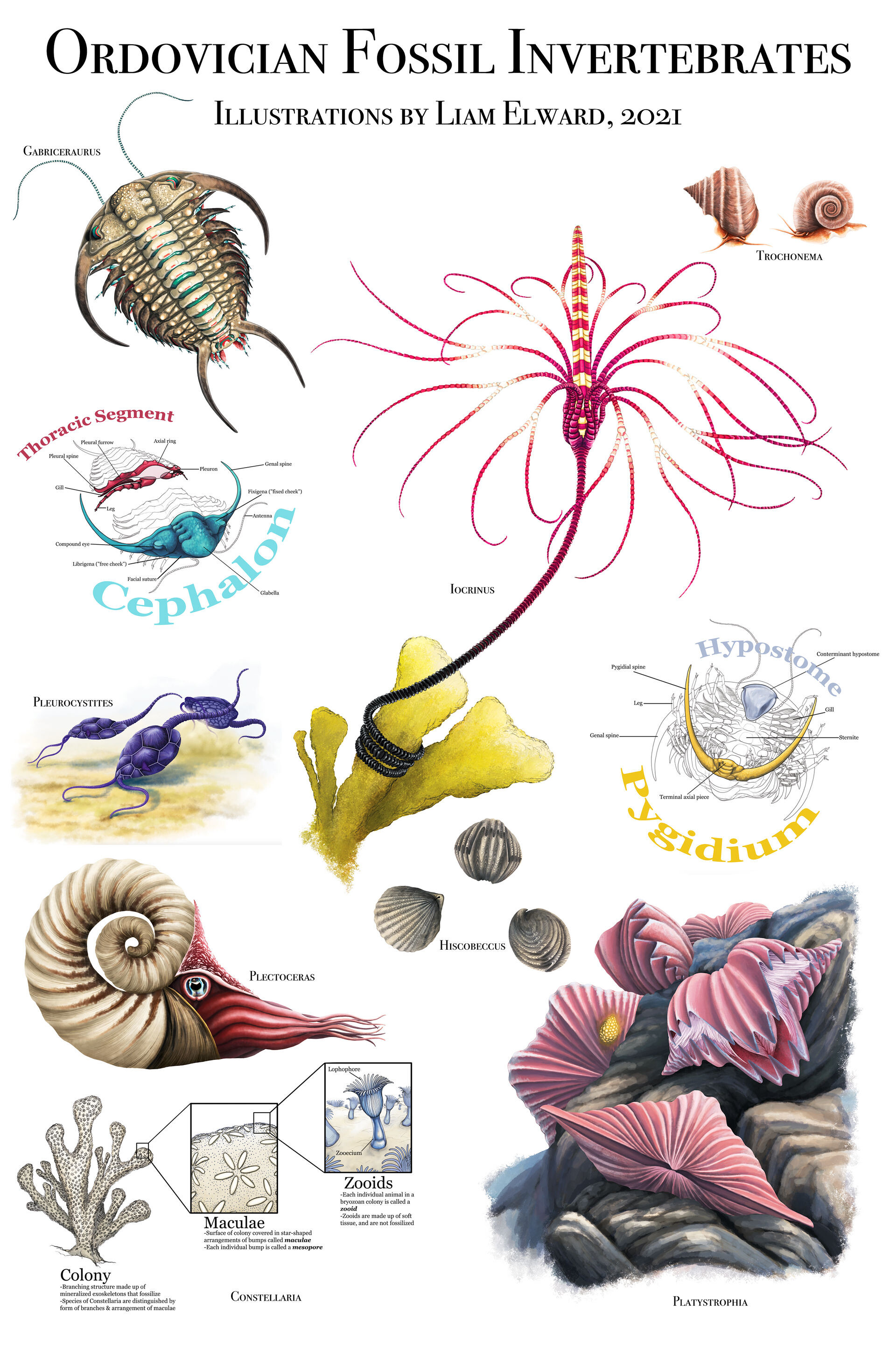The image, resembling a poster, has a plain white background with no visible borders. At the very top, in bold black capital letters, it reads "ORDOVICIAN FOSSIL INVERTEBRATES". Just below, in smaller black print, it states "Illustrations by Liam Elward, 2021". The image features around ten detailed, computer-generated illustrations of various Ordovician invertebrate fossils, each labeled with their scientific names in small black text. 

On the upper left is an organism resembling a scorpion, possibly a Debrisaurus. In the upper right, there are two snail-like illustrations labeled Trachonema. The central illustration features a long, narrow-bodied creature with numerous tentacles, identified as Iocrinus. Below this, a segmented invertebrate displays a red thoracic segment and a blue cephalon (head), with labels indicating "Thoracic Segments" and "Cephalon". 

Further down, clusters of purple, tentacled forms labeled Pleuroscythes are visible. Below this, a squid-like creature with trailing tentacles ending in a curled shell is labeled Pleurosurus. An illustration in the center depicts what looks like a colony, potentially coral, with labels identifying its parts as "Immaculi" and "Zoids". In the lower right corner, pink shells on a rocky cliff are labeled as Platystrophia, and to the left above them are round shells labeled Hiscobicus.

The lower left features a larger pink shell illustration, while to the right, another segmented creature, resembling the earlier scorpion-like figure but with blue and red coloration, is labeled with parts such as "Hippostome" and "Pygdemion". The overall style of the illustrations is reminiscent of those found in educational textbooks, combining visual appeal with scientific accuracy.